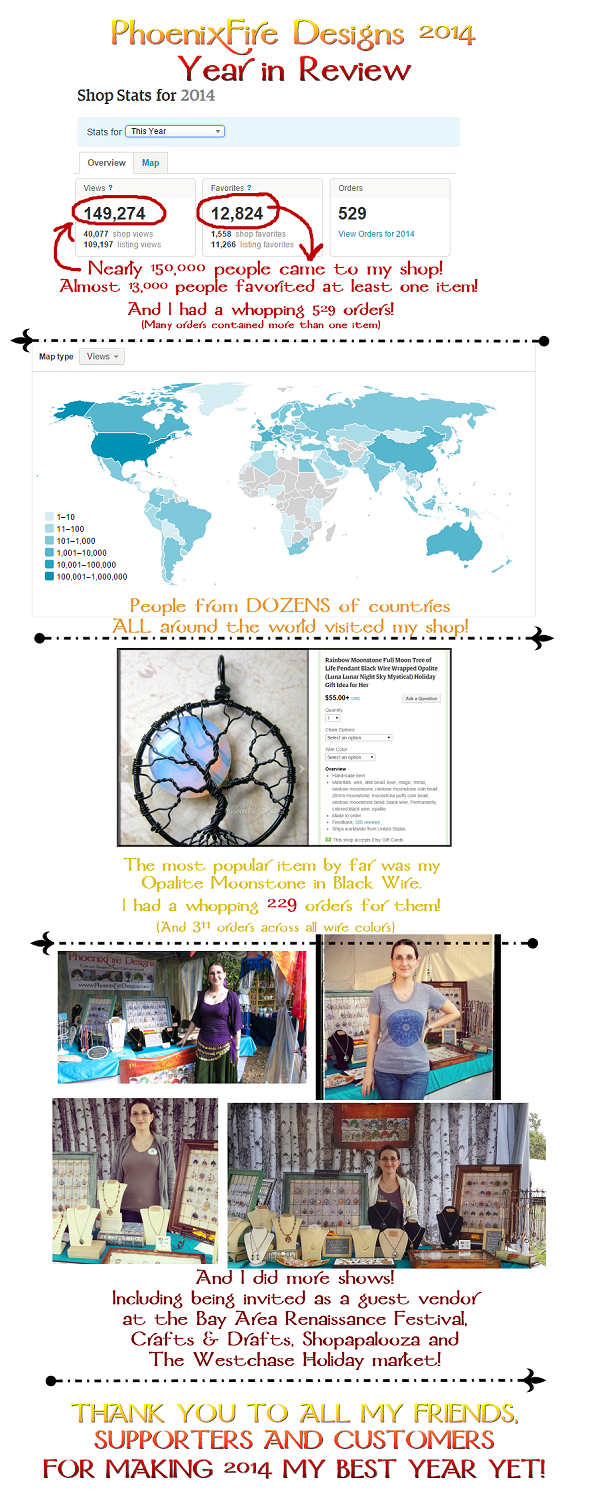**Phoenix Fire Design: 2014 Year in Review**

This image is a comprehensive year-in-review poster for Phoenix Fire Design, a jewelry store—possibly an online retailer—featuring a detailed mix of visuals and statistics. The poster opens with statistics from 2014 in red text: "Nearly 150,000 people visited my shop. Almost 13,000 people favorited at least one item, resulting in an impressive 529 orders, many of which included multiple items."

Below this, geographical outreach is depicted with a world map, creatively shown in a flattened rectangular format. Several countries are highlighted in varying shades of green, indicating the global reach of the shop and the density of its visitors; darker green areas signify regions with more visitors.

At the bottom of the poster, photos showcase the individual behind Phoenix Fire Design, proudly standing next to display cases filled with their jewelry creations. The image concludes with a heartfelt message: "Thank you to all my friends, supporters, and customers for making 2014 my best year yet!"

The blend of graphs, real-life images, and graphical elements paints a vivid picture of a successful and globally recognized year for Phoenix Fire Design.